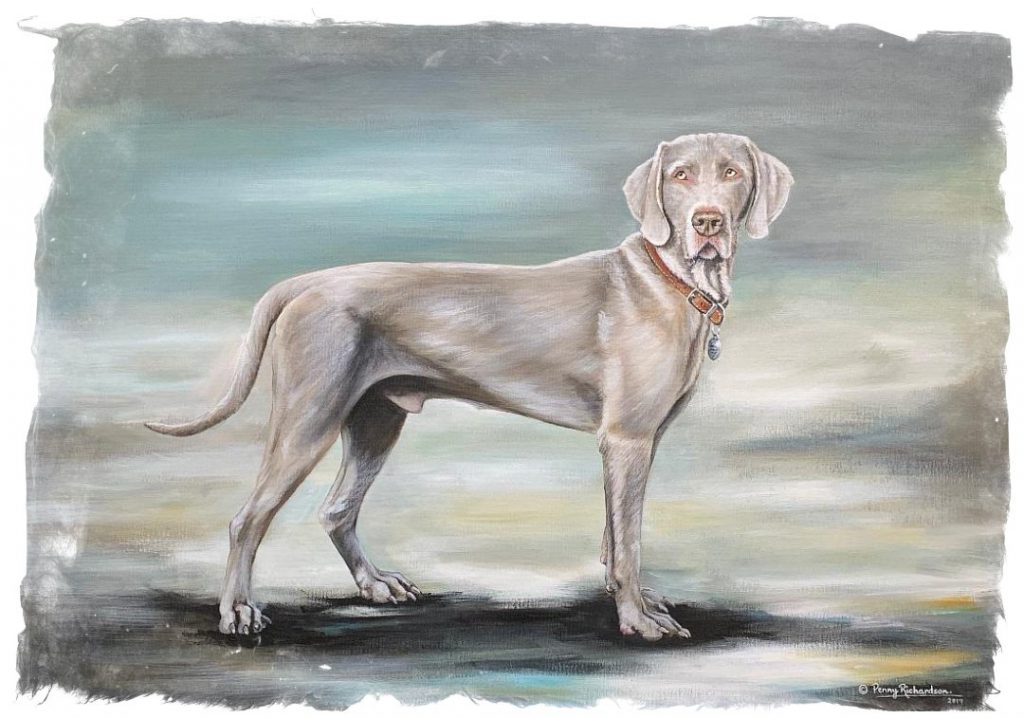The painting features a dog that closely resembles a Labrador retriever or possibly a bloodhound, characterized by its light brown or grayish-brown fur. The dog is shown in a side profile, standing tall with its body oriented to the left while its head is turned to look directly at the viewer. Its facial expression conveys a serious or mournful look, emphasized by darker brown areas under its eyes and a brown nose. The dog’s long tail hangs down and curls slightly at the end. It wears a brown collar adorned with a small dog tag.

The background of the painting features horizontal brush strokes of varying colors and intensities, including teal in the upper left-hand corner, some white, and a surrounding grayish-blue hue, creating a textured and dynamic setting. Beneath the dog, there are hints of blue and orange, possibly suggesting a reflection or a stylized shadow. A distinct shadow cast by the dog adds depth to the image. The artist’s signature is positioned in the lower right-hand corner but remains unreadable due to its small size.